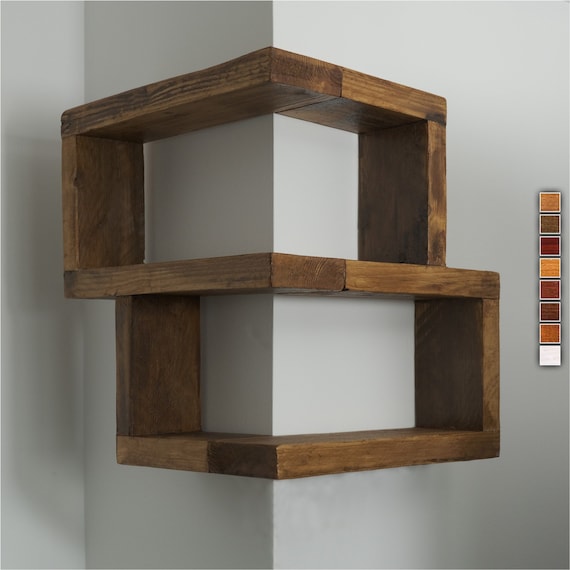This photo showcases a unique and modern corner shelf designed to wrap around the corner of a wall rather than fitting into it. The shelves are made of light brown wood, shaped into two rectangular prisms that are creased in the center to snugly fit the corner, forming a V-shape against the plain white wall. This innovative design creates an optical illusion, as it appears the shelves could be flipped to fit into the corner, but they are specifically made to wrap around it. The top shelf protrudes slightly more than the bottom one, and each shelf offers enough space to display small items like knick-knacks, bottles, or small books. In the background, a color chart is visible, indicating that the shelving unit is available in eight different finishes. This piece of furniture serves as both a functional and decorative addition to any room.